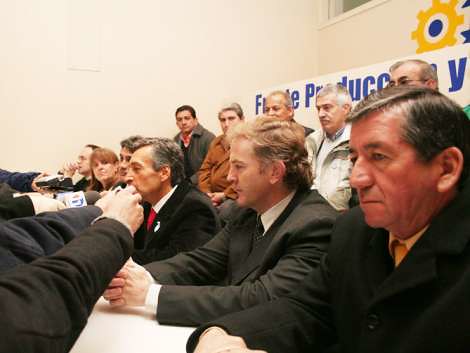This color photograph, captured in landscape orientation, showcases a formal indoor meeting room filled with multiple people. In the foreground, several men are seated in rows, dressed in formal attire—white suits with varying colored ties: one yellow, one black, and one red. The man closest to the viewer, situated on the right side, appears to be in his 50s and is attentively looking towards the left-hand side of the image where individuals with outstretched arms are holding microphones, presumably conducting interviews. 

Behind the seated men is a stark white wall adorned with a white banner featuring dark blue lettering and gear shapes, lending a professional atmosphere to the scene. Further back, another row of attendees is visible, comprising individuals in more casual jackets, including one white and one brown. The background figures seem to be workers or support staff observing the proceedings. The image exemplifies photographic representationalism realism, capturing the detailed interactions and attire of the subjects within this organized setting.